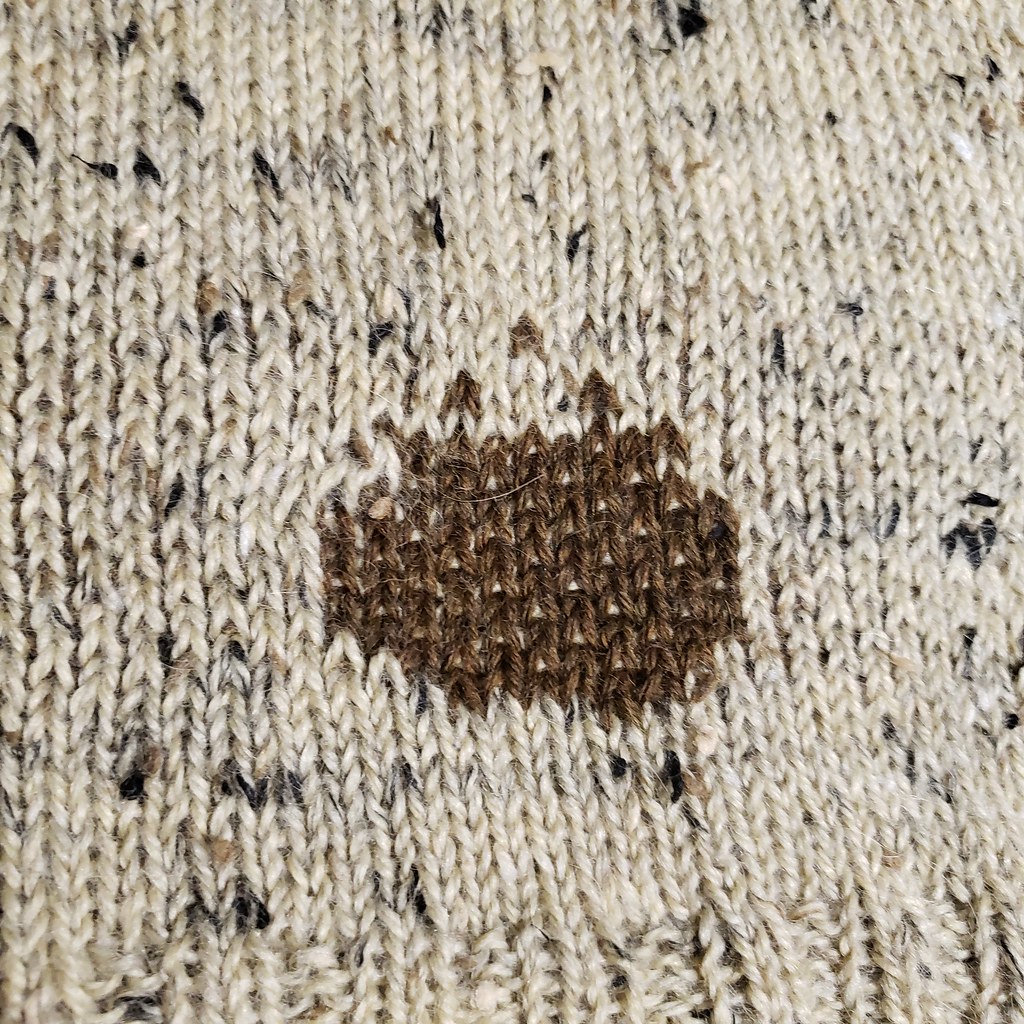The image is a precisely square, highly detailed photo of a knitted fabric piece. The material, likely made of yarn and possibly stemming from a woolen or wool-like origin, features a predominant beige or cream color interspersed with specks of dark brown and black. The fabric is laid flat and in the center lies an irregularly shaped brown area, which stands out distinctly from the rest of the material. The image appears to capture a close-up view, revealing a vertical pattern of V-shaped knit stitches resembling a fishtail, running from top to bottom. The exact nature of the item remains ambiguous due to the close-up nature of the photograph, but suggestions include it being part of a sweater, scarf, or quilt.